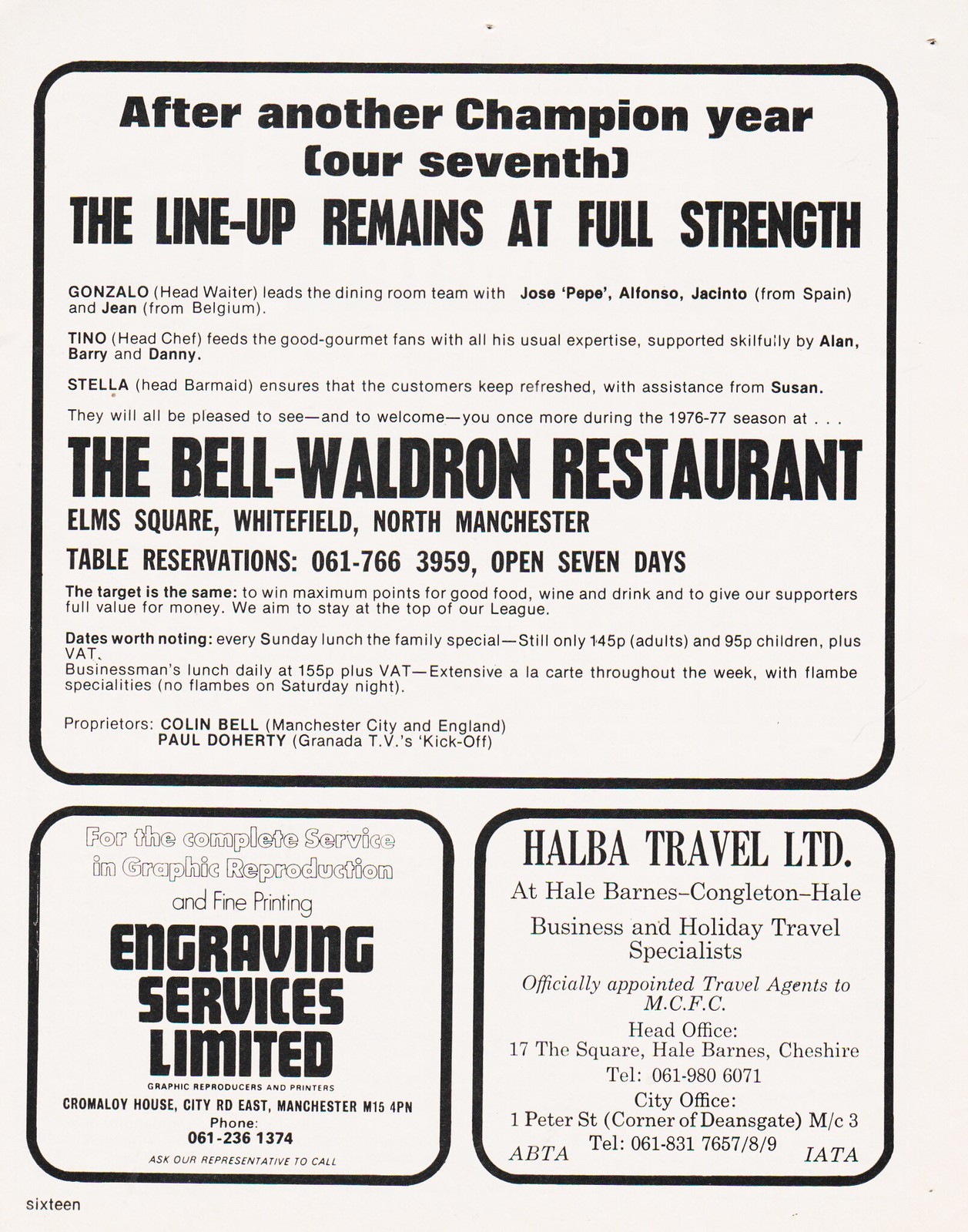The image is a black-and-white printed page, likely from a vintage program or magazine, designated as page 16. It features three distinct advertisements arranged in a portrait orientation, each outlined with dark black rules and rounded corners. The top half of the page is dedicated to an ad for the Bell Waldron Restaurant, celebrating their seventh champion year with the message, "After Another Champion Year (our 7th), the lineup remains at full strength." Underneath, it includes the restaurant's address: M Square, Whitefield, North Manchester, and a phone number for table reservations: 061 766 3959. The lower half of the page is split into two quarter-page ads. On the left, an advertisement for Engraving Services Limited boasts "For the complete service in graphic reproduction and fine printing," followed by their address and contact information. To the right, an ad for Halba Travel Limited highlights it as a consultant for business and holiday travel, based at Hale Grounds. This ad also provides multiple lines of contact details. The overall style of the page is indicative of a vintage print publication.